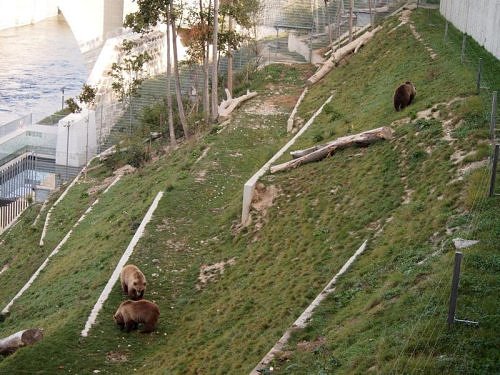This outdoor photograph captures a green grassy hill with an uneven, patchy ground consisting of short green grass interspersed with brown dirt and gray rocks. Three brown grizzly bears roam the hillside; two are positioned in the bottom left corner of the image, with one in profile, appearing to eat something on the ground, while the other bear has its back turned, showcasing its shiny deep brown coat and characteristic hump. The third bear is higher up on the hill towards the top left, its back also facing the camera.

In the top left of the photograph, there is a waterway, possibly a lake or river, which has a blue color with slight ripples. The water is visible just behind some white stone walls. The hill inclines towards the right, where metal poles and wire fences extend from the lower right to the upper right corner. Further up and behind the hill, there are taller fences made of horizontal metal bars. White ledges ascend the hill, providing it with structure. There are also a few exposed tree roots and possible cylindrical pipes emerging from the ground. Additionally, a tall white barrier wall stands prominently in the far upper right, with a few large trees visible near the top of the image. Sunlight can be seen faintly in the background, indicating that the photo was taken during the daytime.